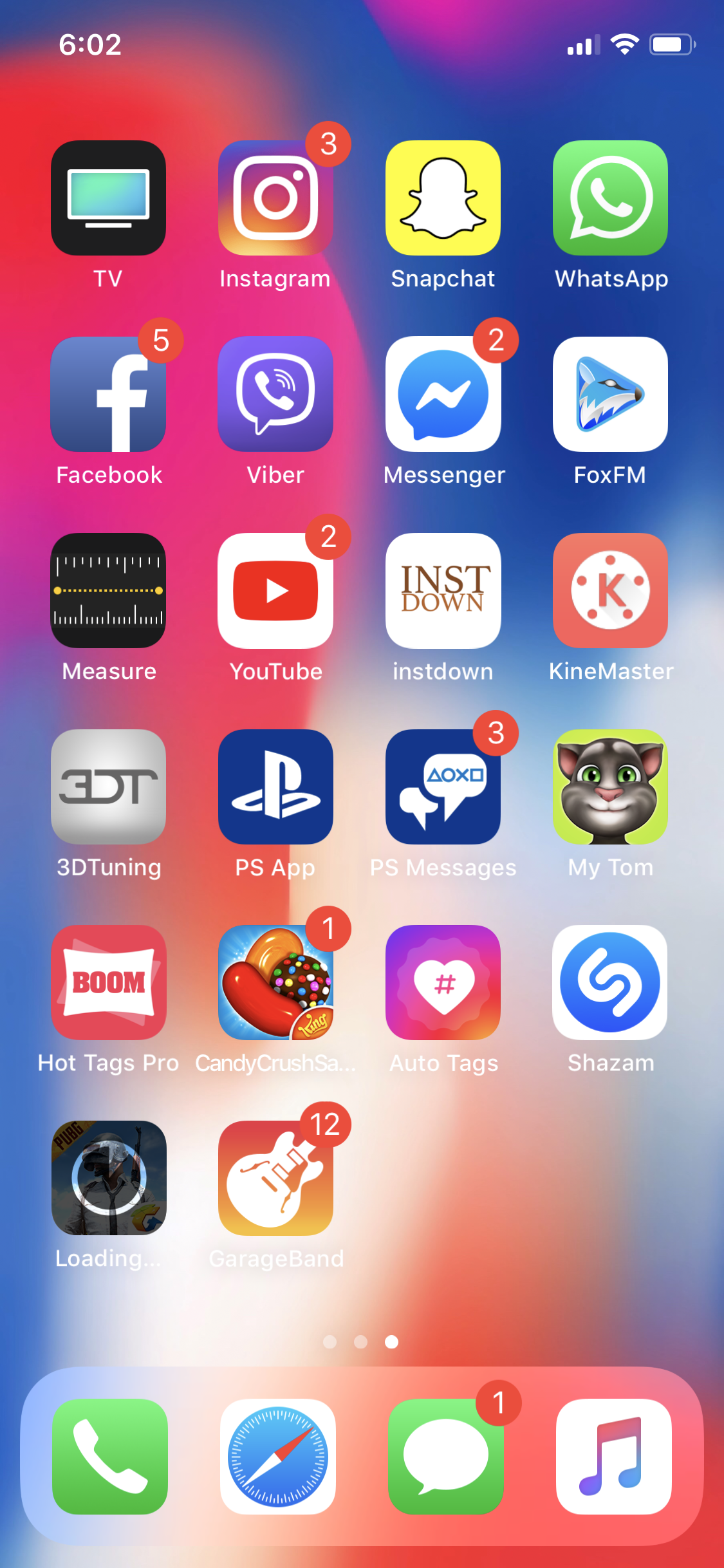Screenshot of a mobile phone's home screen: At the top left corner, the time reads "6:02" with signal strength bars, a Wi-Fi icon, and a battery indicator beside it. The app icons are arranged in a grid format. 

In the top row, from left to right, the apps are: WhatsApp, Snapchat, Instagram, and a TV app. 

The second row, left to right, features: Facebook, Viber, Messenger, and Fox FM. 

Continuing down, the third row includes: Lcollapse, Kine Master, Inst Down (listed as INST Down), and YouTube. 

The fourth row presents: Measure, 3D Tuning, PS App, and PS Messages. 

The fifth row contains: My Tom, Shazam, Auto Tags, and Candy Crush. 

In the sixth row: Hot Tags Pro, Loading, GarageBand, and the Phone App. 

Finally, at the bottom, the dock holds the Safari app, Messages app, and iTunes app.